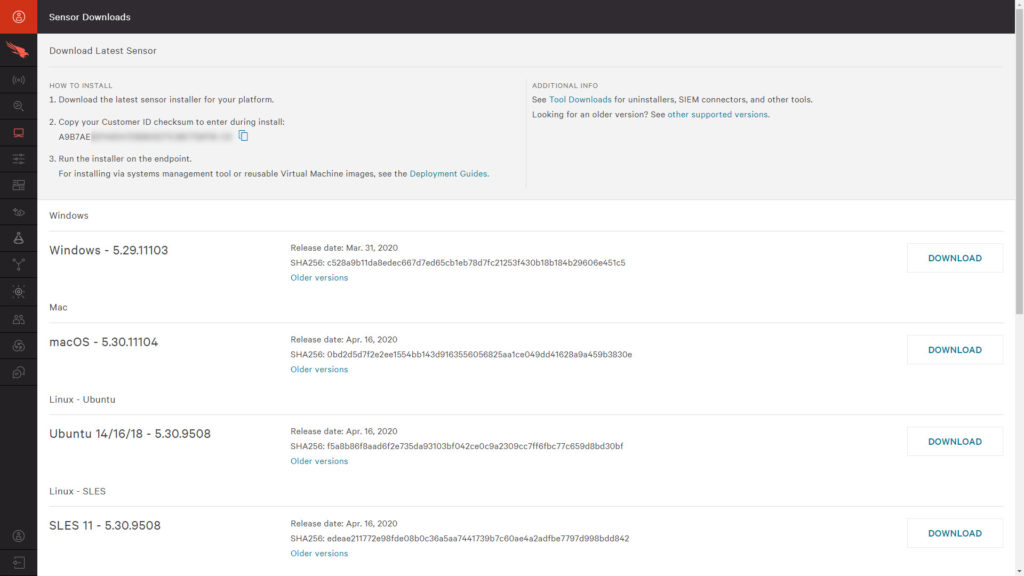This image is a screenshot from a webpage with a challenging-to-read, small font size, but it clearly shows the graphic layout and elements. At the very top, there's a narrow black border. A thin black sidebar appears on the left, with a red square at the top left corner that possibly houses an account page icon. The sidebar contains several faint icons, likely representing utilities such as downloads.

The main section of the webpage has a light gray background in the top quarter and a white background in the remaining three-quarters. At the very top left of this section, there is a header that reads, "Download Latest Sensor." Below this, it instructs visitors on how to download and install: "Download the latest sensor installer for your platform." It also advises users to "copy your customer ID checksum to enter during install," though this instruction is challenging to read due to the font size.

The white section features a headline labeled "Windows" on the left side, listing several Windows versions, though primarily highlighting one. The middle of this section records the release date as "March 31, 2020," and on the right is a button for downloading the software. Beneath the Windows section, the page lists software for "Mac," followed by "Ubuntu," and finally "Linux SLES."